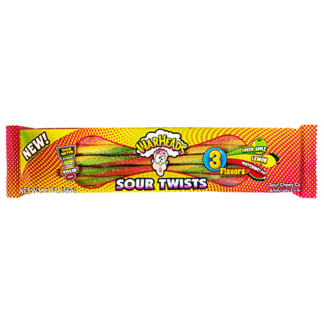The image depicts a long, rectangular package of Warheads Sour Twists candy, designed with a vibrant yellow and red half-tone pattern that gradients out in a wavy fashion towards the edges. The center features a viewport displaying spiral-shaped sticks of candy in red, yellow, and green—representing the three flavors: apple, lemon, and watermelon. The Warheads logo, prominently placed at the center, showcases a cartoon face with a humorous, puckered expression and a mushroom cloud above its head. The word "Warheads" is emblazoned within the cloud in bold yellow text with pink tips at the bottom, while "Sour Twists" is written beneath it in a combination of white and pink text. Additionally, a "New!" label with an exclamation point is situated in the top left corner of the package. The background enhances the playful design with a prominent yellow color complemented by scattered red dots, and an hourglass-like shape on its side, filled with the candy’s vibrant colors.